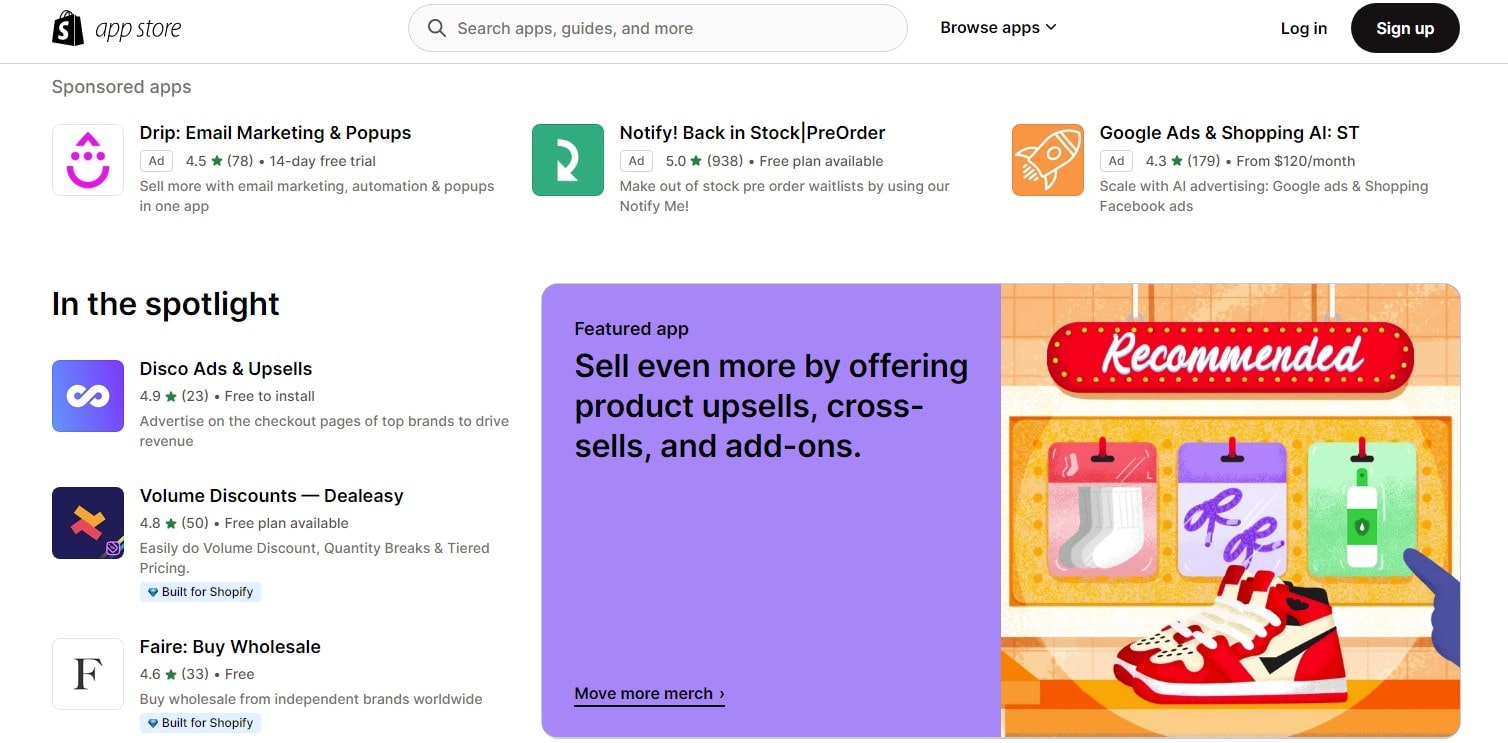Here is a detailed and cleaned-up caption for the image:

---

The image is a screenshot from a website with a clean, white background. At the top left corner, there is an icon of a shopping bag with an 'S' on it, immediately followed by the text "App Store." Moving to the right, there is a search bar next to the "Browse Apps" option. On the far right, there is a "Login" button, accompanied by a prominent black circle with the text "Sign Up" in white lettering.

Below this top bar, there is a section titled “Sponsored Apps.” It features various app names such as Drip, Email Marketing, Pop-Up, Notify, Backup, and Stock Pre-Order, alongside Google Ads and Shopping.

On the left-hand side of the image, there is a section titled "In the Spotlight," listing Disco Ads and Upsells, Volume Discounts, and Faire by Wholesale.

Towards the middle-bottom of the image, there is a purple square labeled "Featured App" with the message: "Sell even more by offering products, upsells, cross-sells, and add-ons."

To the right of this purple square, there is an image of a pair of shoes with a finger pointing towards a picture of a bottle. Below this image, there is another black circle with "Recommended" written in white letters.

---